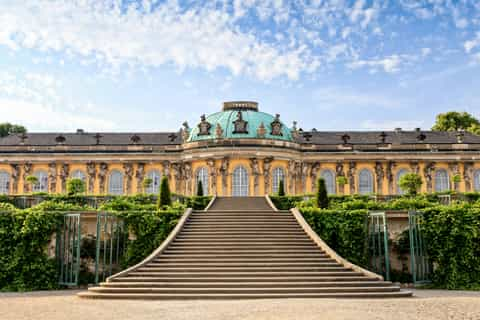The image showcases a grand European-style building that exudes an Austrian architectural influence, potentially placing it in Vienna, Austria. Dominating the scene is a massive, ornate yellow building with rich decorations and multiple arched windows, each surrounded by greenery. The structure appears to be two to three stories high, resembling a grand hotel with expansive balcony walkways.

A central feature of the image is a large, sweeping staircase that splits into two paths, leading up to the imposing domed roof in the middle of the building. This dome, adorned in a minty seafoam green or turquoise color, is topped with golden circular objects and possibly crosses, contributing to its regal appearance. Flanking the staircase are rusted, open gates and lush greenery, adding to the picturesque scene.

The overall composition is completed by a bright, clear blue sky with scattered white clouds in the background, enhancing the majestic and serene atmosphere of this captivating architectural marvel.